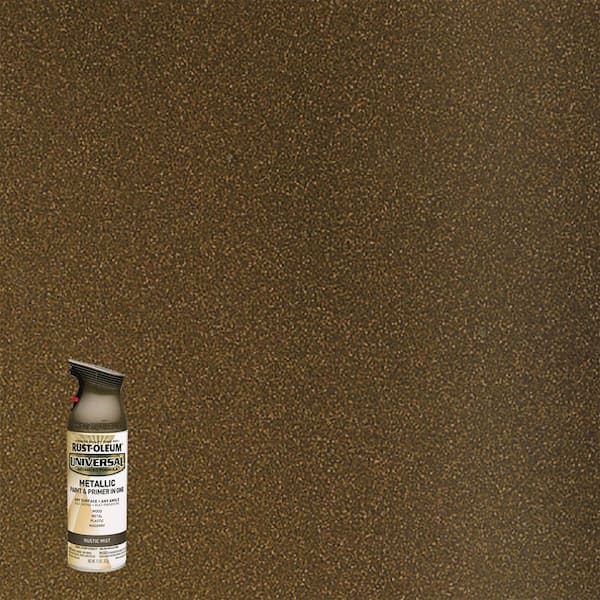A square image features a mainly brown, textured background that resembles a rust-colored metallic surface with light and dark speckled patterns. This texture possibly represents a surface treated with the product depicted in the same image. In the bottom left corner, occupying about an eighth of the total image size, is a spray canister. The canister is white at the bottom with a black top and a red spray nozzle. It is labeled "Rust-Oleum Universal Metallic Paint and Primer in 1" in black text, with additional, smaller text that is unreadable. This image likely serves as an advertisement or description for the Rust-Oleum product, showcasing the color and texture it can achieve.